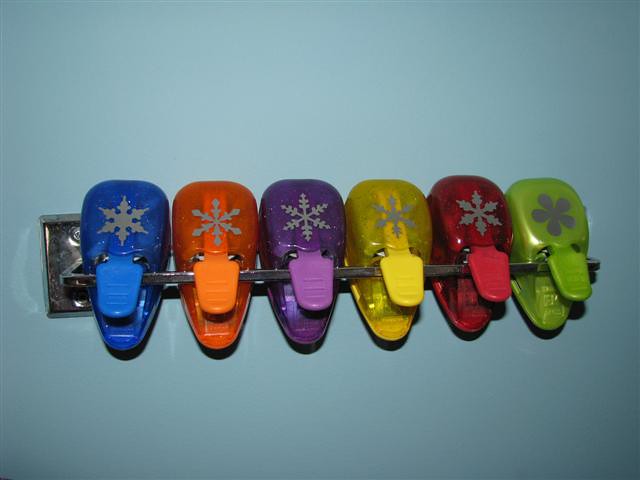The photo captures a set of six colorful decorative hole punchers clipped onto a sleek, chrome towel rack against a blue wall in a bathroom setting. The hole punchers, arranged in a neat line from left to right, are blue, orange, purple, yellow, red, and green. Each puncher, except the green one, which has a flower design, features a unique snowflake pattern. The red and yellow punchers share the same snowflake style, while the blue, orange, and purple each display distinct snowflake designs. The punchers, sparkling slightly, are attached by their thumb press levers hooked over the edge of the rack. The green puncher differs slightly in translucency and possibly shape, adding a unique touch to the uniform line-up of vibrant, whimsical snowflake designs.